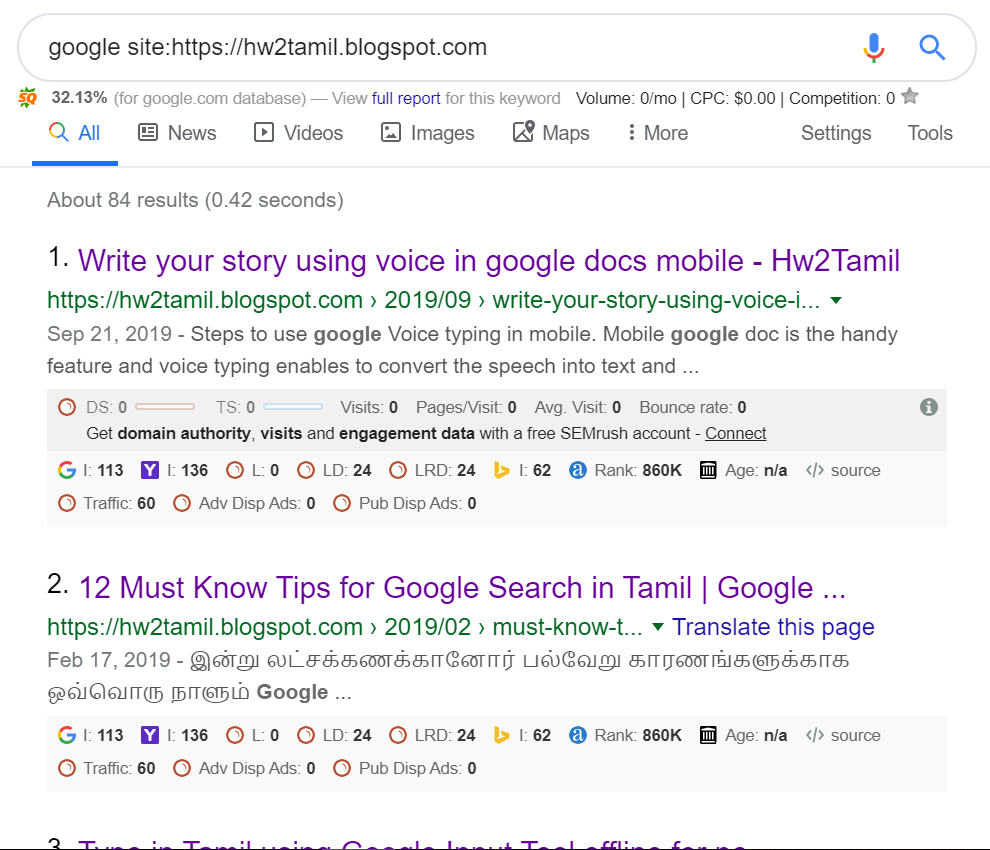This image is a close-up screenshot of Google search results. At the top, the search bar contains the query "Google site: https://hw2tamil.blogspot.com." Below that, a section displays the following information: "32.13% for Google.com database" and an option to "View full report" for this keyword, where "full report" is a clickable link. Additional stats shown include "Volume: 0/mo," "CPC: $0," and "Competition: 0."

The visible search results show two complete entries and the very top of a third result. The first result is titled "Write Your Story Using Voice in Google Docs Mobile" followed by the site name "hw2tamil.blogspot.com."